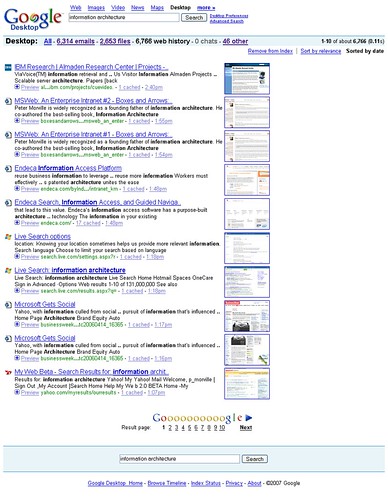The image depicts an interface of Google Desktop, showcasing various features including Web, Images, Video, News, Maps, and Desktop, with the "Desktop" tab selected in black while the others are highlighted in blue. The interface displays a summary of searches: 6,314 emails, 2,653 files, 6,768 web history records, 0 chats, and 48 other items, all sorted by date.

A list of website hyperlinks is prominently displayed on the left side, accompanied by preview thumbnails to the right. The bottom section features a classic Google search results page with pagination from 1 to 10, where the number "1" is currently selected and lacks an underline, unlike the other numbers. The "Next" button and a search bar are situated at the bottom, facilitating easy navigation and further searches.